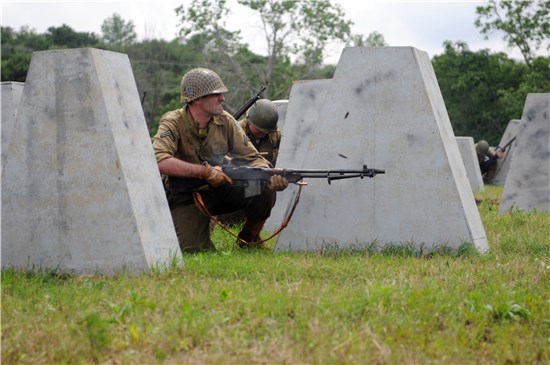In this outdoor daytime photograph, three soldiers in military gear are captured in the midst of a tense scene, likely a historical reenactment of a Vietnam or World War II era gunfight. The image, rectangular and approximately three to four inches in width and two inches in height, features a lush green and brown grassy terrain providing cover for the soldiers.

Foregrounded to the left, a soldier is prominently kneeling behind a trapezoidal stone barricade. These light gray, cement-looking structures have their tops cut off and appear to be nailed together, hinting at a potential wooden construction. The soldier wears a green helmet with mesh netting, a light tan shirt with sleeves rolled up to the elbows, and greenish-gray pants. He sports gloves that are either blue or brown. With a strained, angry expression, he fires a long rifle, its strap hanging down, while bullet casings fly mid-air around him.

To the right, partially obscured by the barricades, another soldier is visible reloading his weapon, closely followed by a third soldier in the distant background. All three wear matching green helmets. The backdrop reveals a clear, blue sky above a canopy of green trees, accentuating the dire situation amidst the calmness of nature.